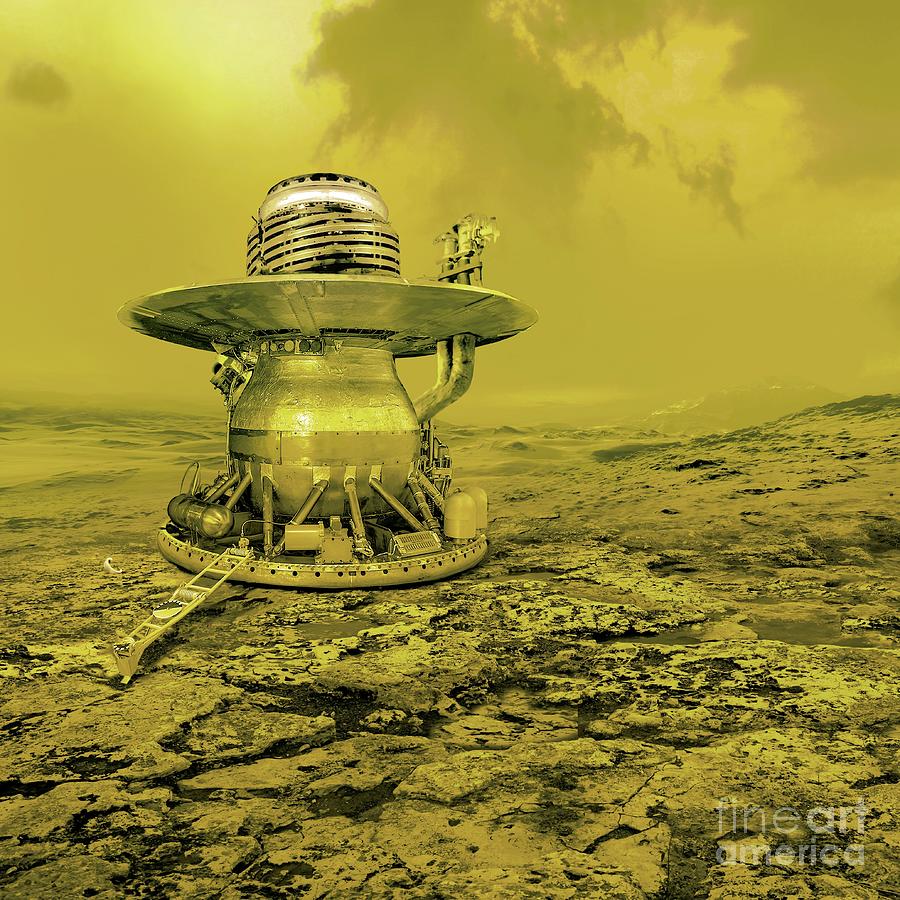This image presents a stark and futuristic barren landscape, predominantly tinted in a monochromatic yellow hue. It appears to be of a desolate, otherworldly terrain, featuring a central, silver-colored machine that resembles a lander or an exploratory vehicle that might be used on another planet. This machine, characterized by its numerous valves, attachments, and a large disc in its middle, sits slightly left of center. The ground is cracked and nearly devoid of any plant life, marked with rocky, scaly textures. Hazy clouds fill the sky, blending into the thick mist that obscures the distant mountainous backdrop. The lower right corner of the image contains a watermark reading "Fine Art America." The overall scene evokes a sci-fi aesthetic, with its unclear atmospheric conditions and distinctly alien feel, yet it's ambiguous whether the image depicts something real or a computer-generated simulation.